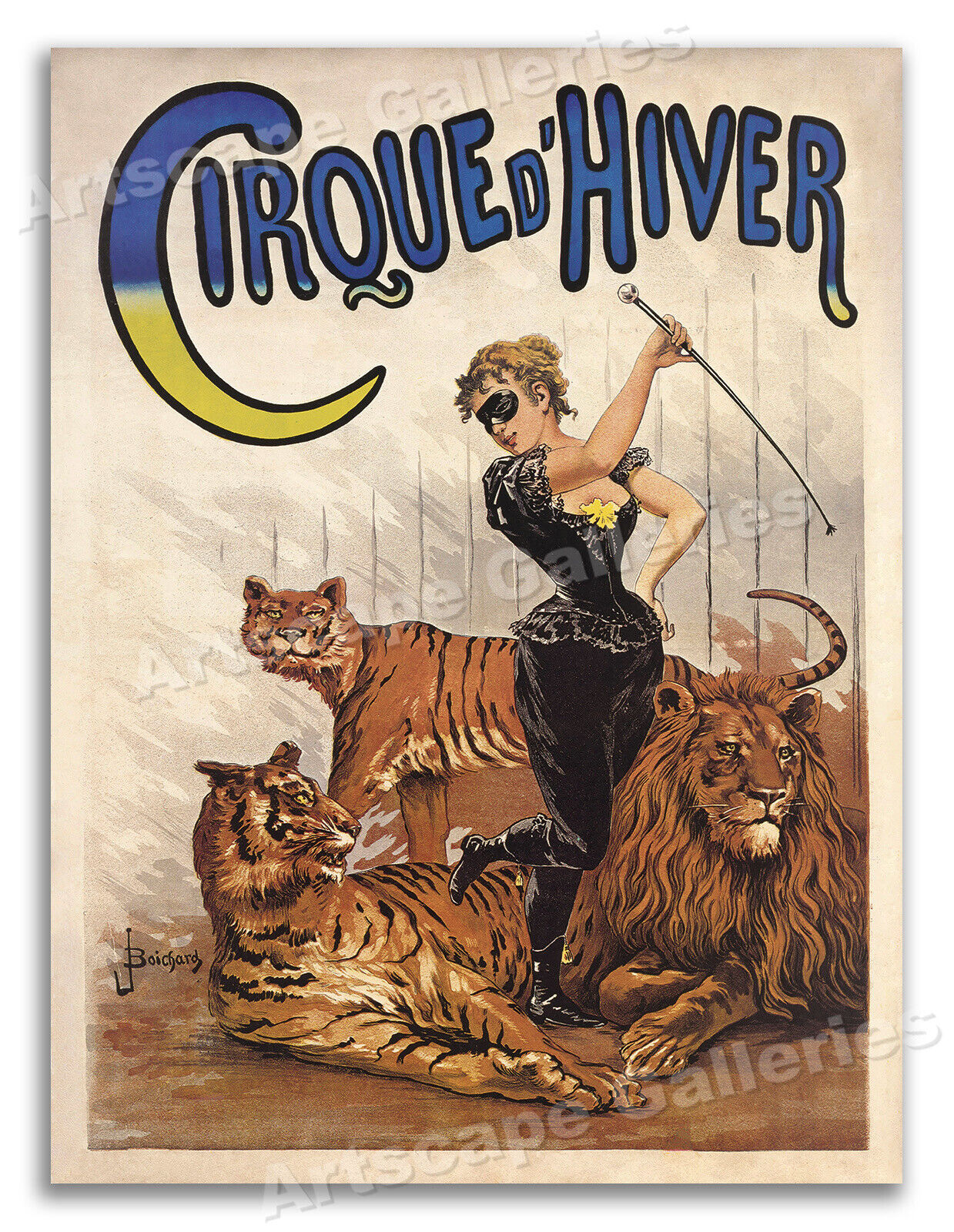A vintage circus poster features prominently the name "Cirque du Verre" displayed in bold, blue letters at the top. A watermark reading "Artscape Galleries" spans across the image, indicating the source of this nostalgic piece. The illustrated scene captures a thrilling moment inside a cage, with sturdy bars visible behind. On the dark brown ground, two majestic tigers and a regal lion appear nonchalant as they lounge. At the center of this tableau stands a poised woman, characterized by her wasp-waisted figure and a dramatic low-cut jumpsuit. Holding a whip in one hand and wearing a mysterious mask across her eyes, she strikes a coquettish pose with one leg flirtatiously raised. Despite the potentially tense scenario, the big cats exude a sense of indifference, adding to the intrigue and allure of this old-fashioned circus advertisement.